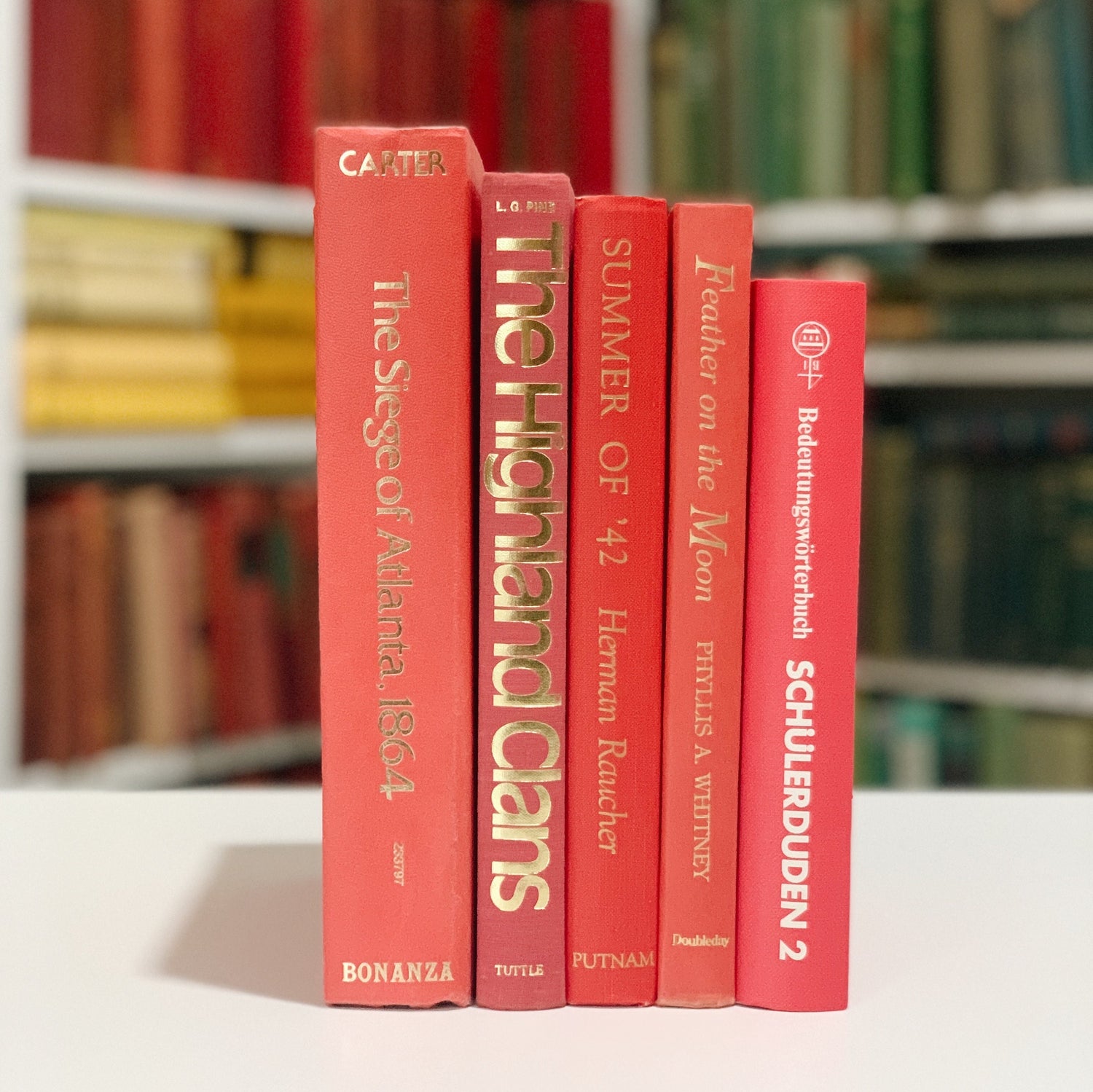This image is a close-up of the spines of five red-covered books, all standing upright on a white surface, likely a desk or counter. The books are arranged from tallest to shortest, starting with the thickest book on the left. The titles, in gold print on the spines, are "The Siege of Atlanta, 1864," followed by "The Highland Clans," "Summer of '42" by Herman Raucher, and "Feather on the Moon" by Phyllis A. Whitney. The fifth book, written in a different language, has white text on its spine. In the blurred background, two bookshelves flank the books, one on the left containing red, yellow, and variously colored books, and the one on the right mostly filled with green books.